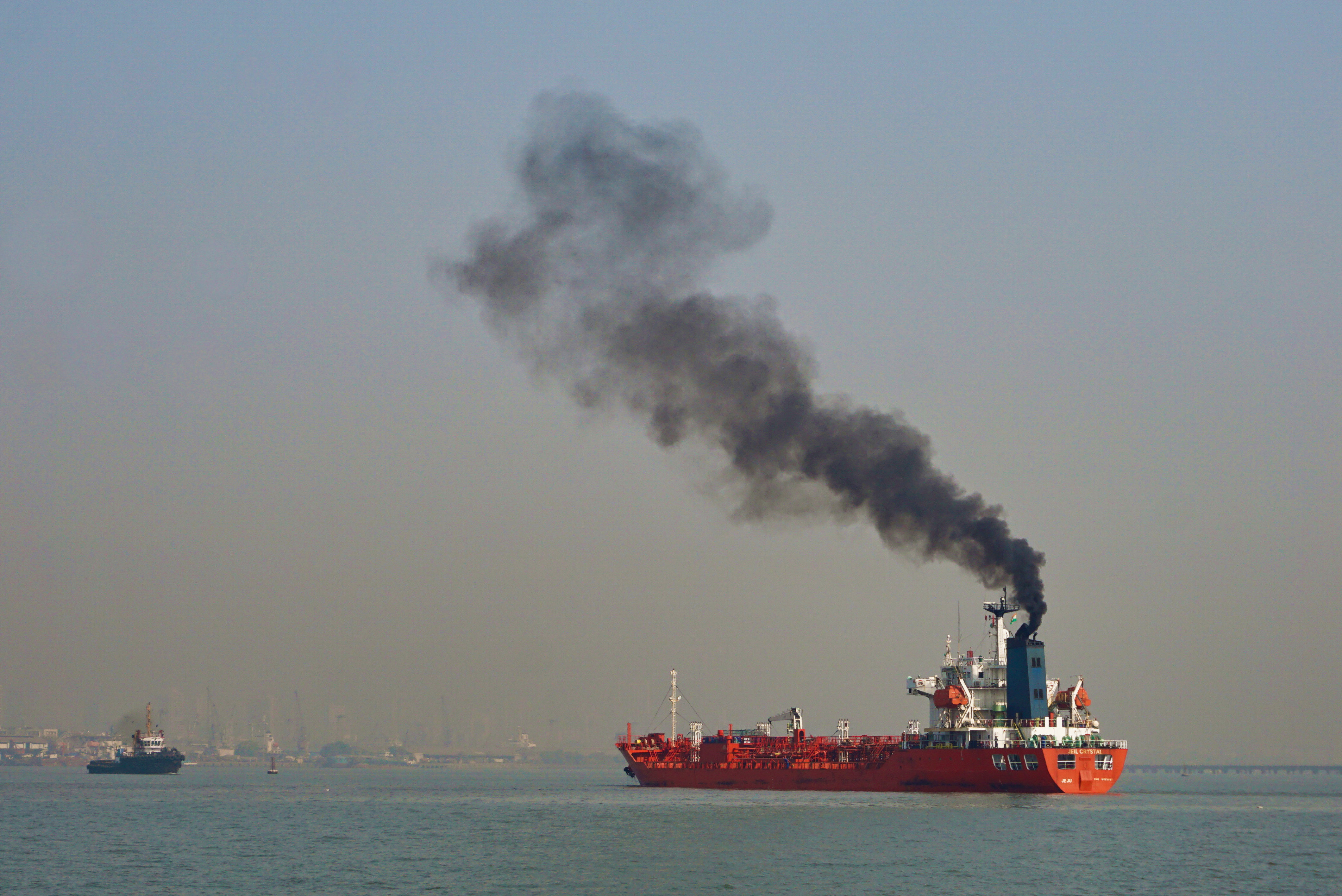The image captures the vast expanse of a calm, dark blue ocean under a gray, cloudy, and foggy sky. Dominating the scene is a large red cargo ship positioned slightly to the right of center. The ship features a tall white superstructure with a blue cabin, from which thick black smoke billows upward, gradually dissipating as it ascends. The vessel is equipped with a white crane and tower-like structures on its deck. To the left of the red ship, closer to the center, is a smaller vessel with a black hull and a white cabin. The foggy background suggests the presence of additional ships, barely visible through the mist. The overall atmosphere is one of deep oceanic stillness and subdued, moody colors.